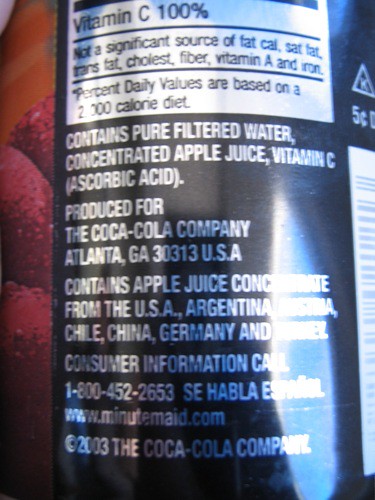This close-up, somewhat out-of-focus photograph showcases a black and silver nutrition and ingredient label on a shiny can. The label prominently states "Vitamin C 100%" and clarifies that it is not a significant source of fat, calories, saturated fat, trans fat, cholesterol, fiber, vitamin A, and iron. The percent daily values are based on a 2000 calorie diet. Further information indicates that the can contains pure filtered water, concentrated apple juice, and vitamin C, along with sorbic acid. The product is produced for the Coca-Cola Company, Atlanta, Georgia, 30313 USA, with apple juice concentrate sourced from the USA, Argentina, Chile, China, and Germany. The label also includes consumer information with a contact number 1-800-452-2653 and a Spanish translation “Se habla español,” along with the website www.minutemaid.com. There is a bright reflection on the side of the can that obscures some of the text, and a barcode is visible on the label. To the left of the black label, there is an orange area at the top and some red-colored berries at the bottom which are very zoomed-in and blurred.